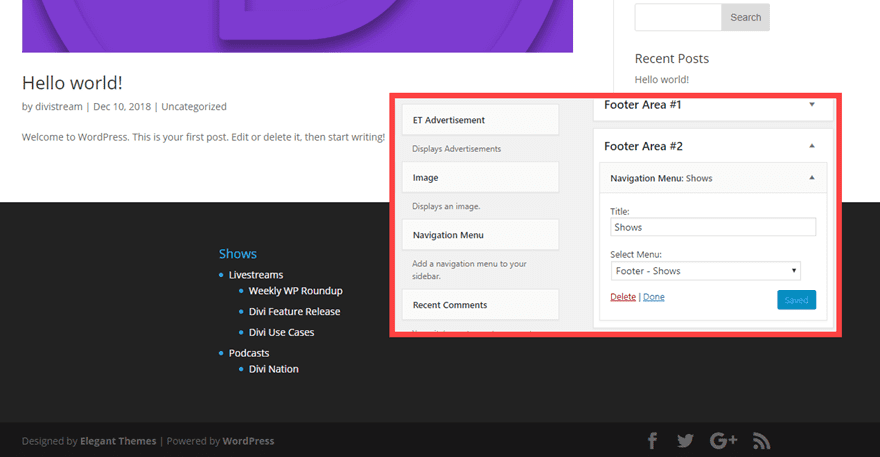The image features a screenshot of a WordPress website. In the background, you can see the main section of the website, which includes a large black footer area at the bottom. This footer contains various options such as Shows, Live Streams, Weekly WP Roundup, Divi Feature Release, Divi Use Cases, a Podcast, and Divination.

Above the footer, there is a section with a white background displaying the text "Hello World by Divstream," dated December 10, 2018, under the category "Uncategorized." The text continues with a welcome message to WordPress, indicating that this is the first post and prompting users to edit or delete it to start writing.

In front of this main background, a smaller box is highlighted with a red border, emphasizing another part of the website. On the right side of the highlighted box, there is a small window displaying "Recent Posts" along with a search bar. At the top of the section containing the welcome message, there is a purple image, which is not fully visible in the screenshot.